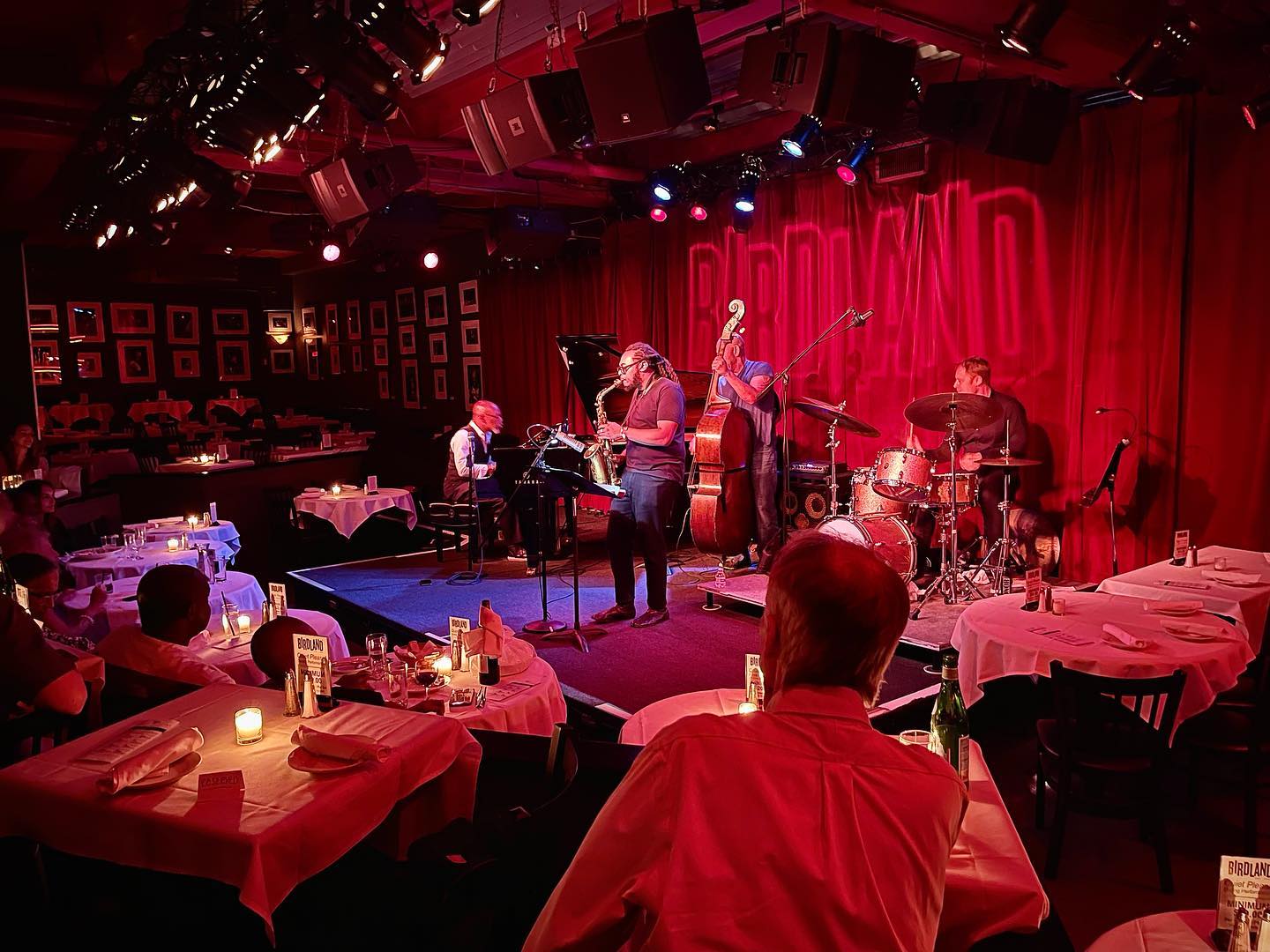The image captures an intense performance by a jazz band at Birdland, with the stage framed by a vivid red curtain featuring the Birdland name in prominent, black-bordered red letters. Central to the scene is the saxophonist, an African-American man with long dreadlocks, who is energetically playing a tenor saxophone while dressed in a short-sleeve shirt and jeans. Next to him is the pianist, and behind them are the upright bass player and the drummer, who sports a long-sleeve shirt, all deeply immersed in their music. The surrounding room is adorned with numerous framed photographs on the walls, extending particularly far down the left side. Below the stage, empty tables with pristine white tablecloths, napkins, and candles are scattered around. In the immediate foreground stands a man, identifiable by his bald patch and white collared shirt, watching the performance with rapt attention. The room has a mix of occupied and vacant tables, indicating a somewhat sparse audience, yet a few patrons sit engrossed, possibly enjoying drinks as they take in the vibrant jazz music.